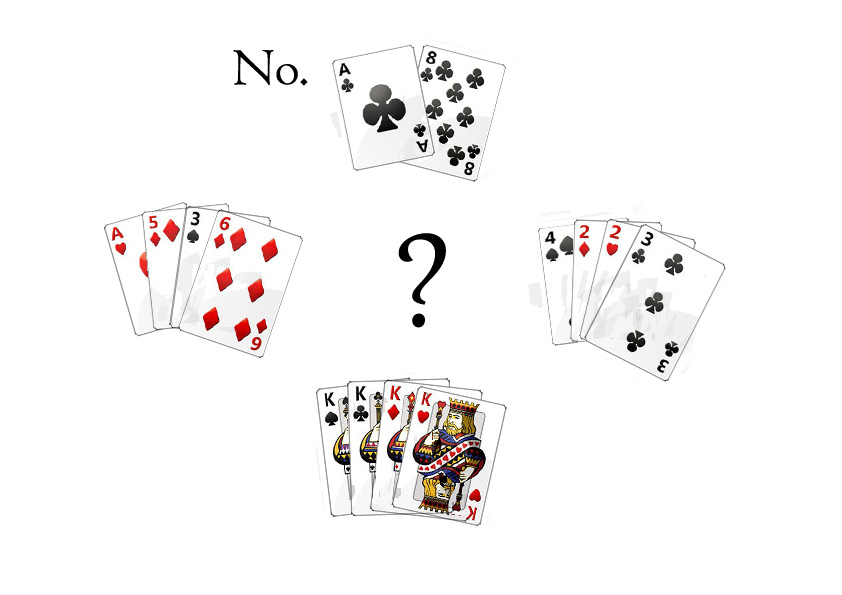The image is a digitally created, minimalist illustration set against a white background. It features four distinct stacks of cards arranged symmetrically, with a black question mark centered in the middle of the arrangement. 

- **Top Stack:** The top stack displays the Ace of Clubs positioned above the Eight of Clubs.
- **Right Stack:** The right stack showcases the Four of Spades, Two of Diamonds, Two of Hearts, and Three of Clubs, arranged vertically.
- **Bottom Stack:** The bottom stack contains all four Kings (King of Spades, King of Clubs, King of Diamonds, and King of Hearts) lined up horizontally.
- **Left Stack:** The left stack presents the Ace of Hearts, Five of Diamonds, Three of Spades, and Six of Diamonds in a vertical formation.

In the upper left corner near the top stack, the word "No." is written in a simple black font with a capital "N" and a period at the end. The illustrations are simple with slight shadows under each stack to give a subtle depth, but otherwise, the design is quite flat, adhering to a standard playing card appearance with white backgrounds and neatly visible suits and numbers.